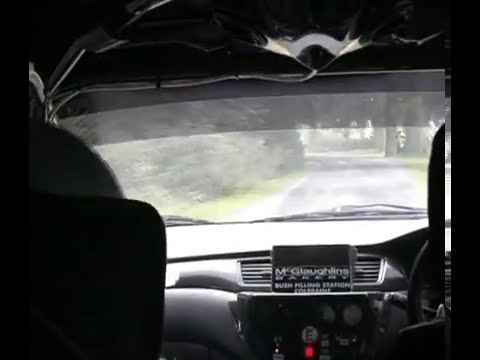The photograph, taken from the backseat of a vehicle, captures the interior and the view through the front windshield. The dark gray and black interior of the car features a central console with various buttons, gauges, and a prominent electronic touchscreen tablet propped up against the two front air conditioning vents. The tablet displays the text "M Glowing" against a black background. The driver is seated on the left side of the car. Outside the windshield, a gray country road stretches ahead, flanked by green grass and lush trees on both sides, creating a serene, countryside setting.